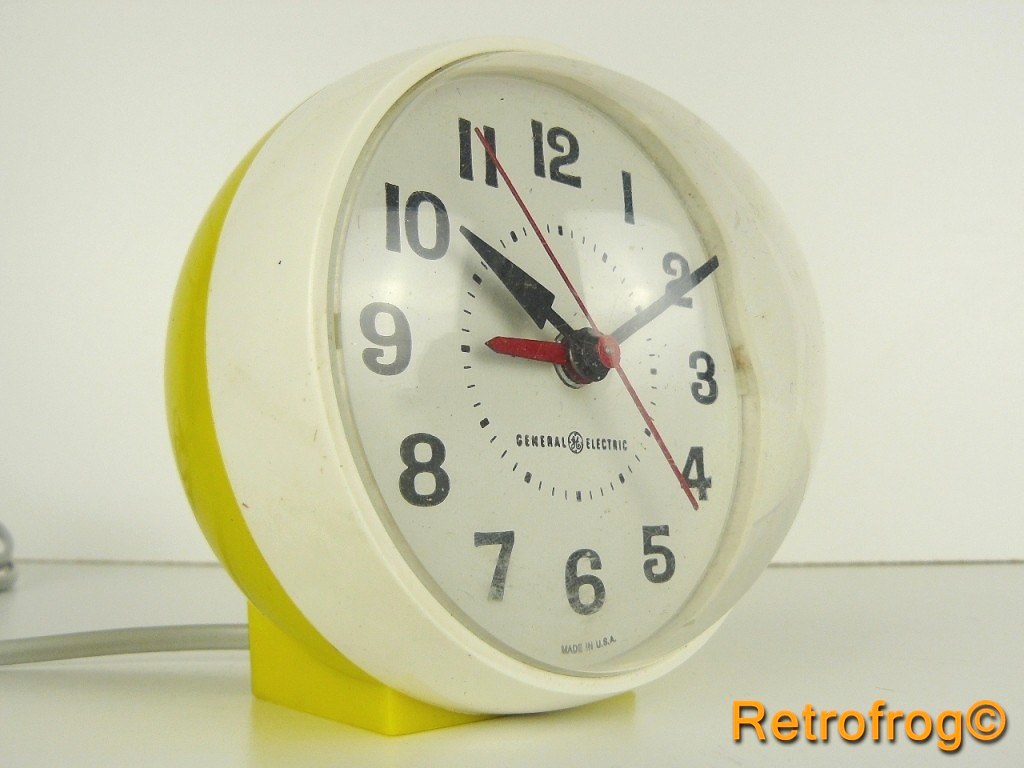This image showcases a classic analog desk clock with a distinct retro aesthetic. The clock features a white face dial, prominently displaying bold black hour and minute hands, complemented by a slender red second hand. Numerals ranging from 1 to 12 encircle the dial, replacing the traditional hour markers. Centrally positioned beneath the hands, the manufacturer's name, "General Electric," is meticulously printed, while at the bottom of the dial, "Made in USA" denotes the clock's origin. Encircling the round clock face, a white outer edge provides a clean contrast to the design. The rear of the clock and its sturdy base are both colored in a light green hue, enhancing its vintage charm. The clock face is protected by a protruding, semi-circular plastic glass case, giving it a dimensional, bubble-like appearance. Adding to its authenticity, a copyright mark from "Retro Frog" is visible at the bottom right of the image.